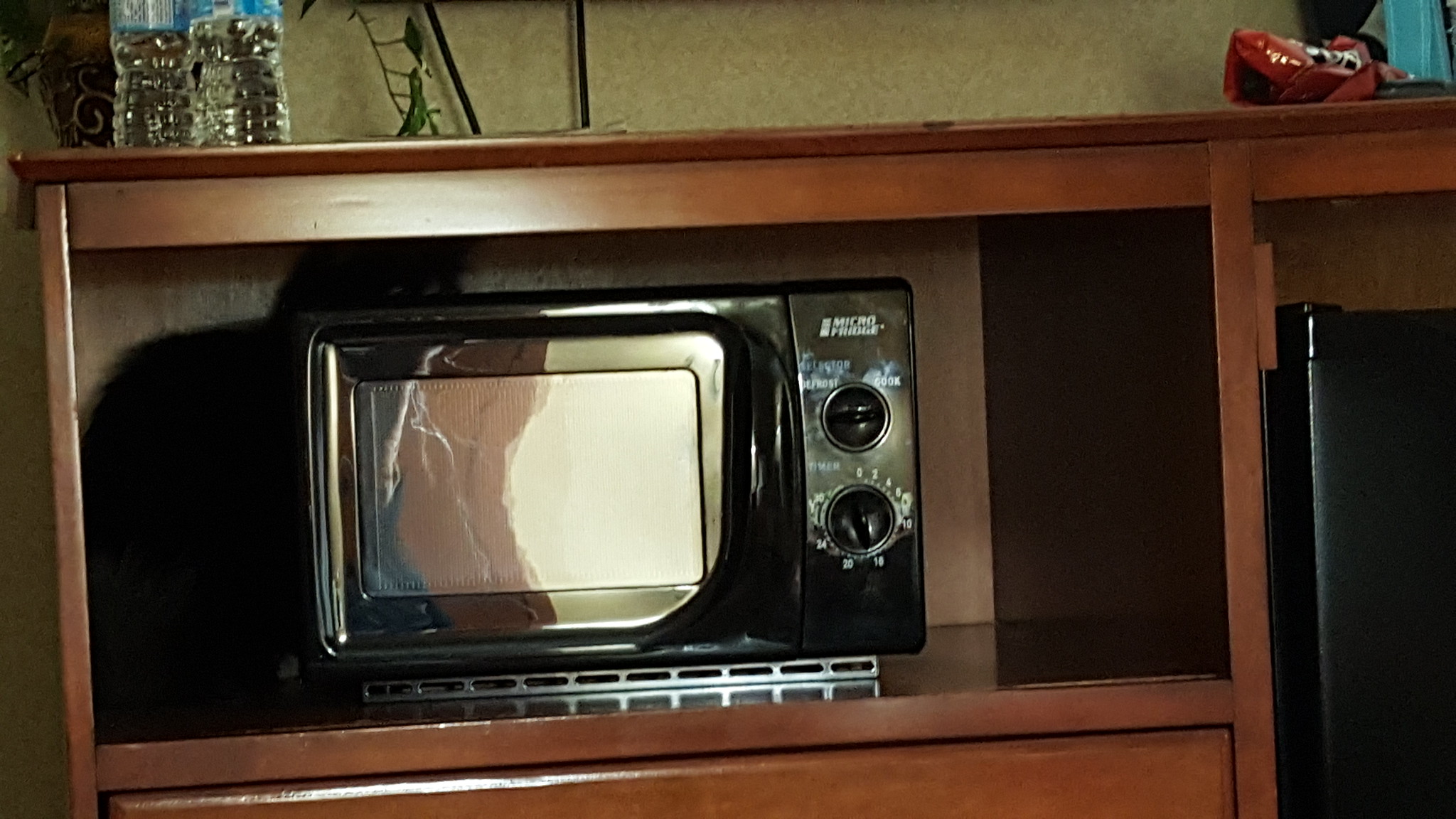The image depicts a hotel room corner featuring a small, black "MicroFridge" microwave integrated within an open shelf of a medium brown wooden cabinet. The microwave, which has a reflective glass window, is equipped with two black dials: the top dial labeled "Defrost" and "Cook," and the bottom dial surrounded by numbers. Above these dials, the brand "MicroFridge" is written in white. Positioned next to the microwave on the right is a small, hotel-sized black refrigerator. Above the microwave, on the countertop, there are two bottles of water with blue labels, a plant with a vine slightly visible, and what appears to be a crinkled brown wrapper with a black design. The entire setup is against a light yellowish wall, and the shadow and reflection of the person taking the picture can be seen on the microwave’s glass window.